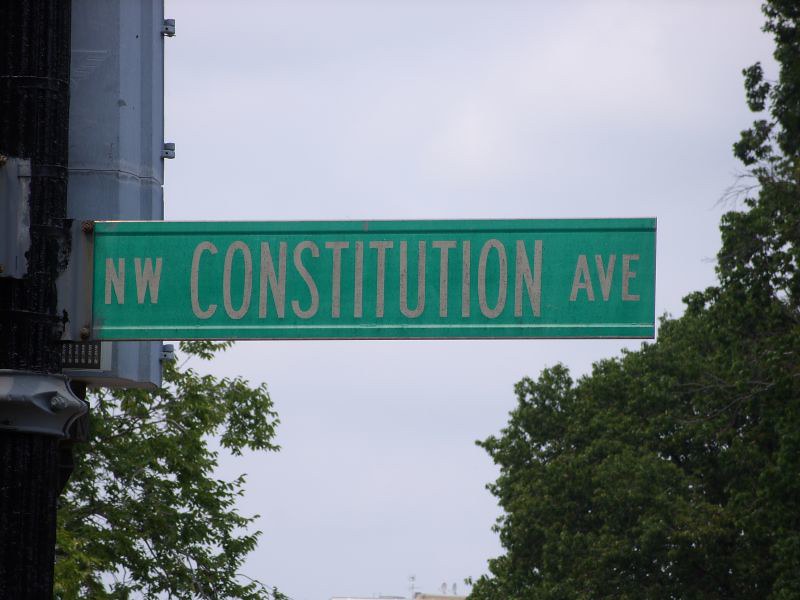In this outdoor image, the primary focus is a rectangular, green street sign situated in the foreground. The sign, which reads "NW CONSTITUTION AVE" in somewhat dirty, white capital letters, is the central element of the composition. The street sign is mounted on a dark-colored pole, which occupies the left side of the image.

In the background, the right side features dense trees with dark green leaves, stretching from the bottom to the top of the frame. A similar tree, also with dark green foliage, is located just below the street sign, adding to the greenery. The sky forms the backdrop, displaying a light bluish-gray shade. Near the very bottom center of the image, there is a barely visible brown rooftop, hinting at nearby buildings. The sign itself is attached to a gray section at the top, completing the structural details of the scene.